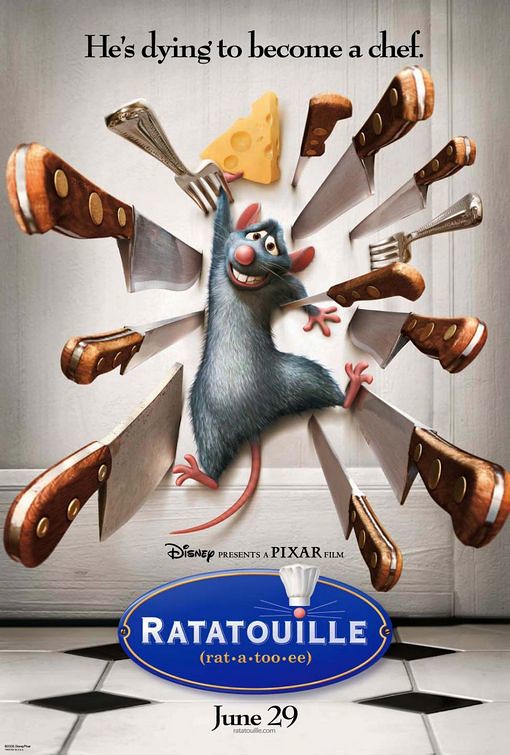This detailed movie poster for the Pixar and Disney film "Ratatouille" features a grayish-blue cartoon rat pinned against a white wall with black diamond-patterned flooring visible at the bottom. Across the top of the poster, a quote reads, "He's dying to become a chef." The rat is surrounded by a chaotic array of butcher knives and forks embedded into the wall, clearly thrown towards him but missing their mark. Above the rat, a piece of cheese dangles, just out of reach. Below, the poster announces, "Disney presents a Pixar film," followed by the stylized title "Ratatouille" featuring a chef’s hat accentuating the 'i' with a rat's nose and whiskers. The word "Ratatouille" is also presented with correct syllabic pronunciation. At the bottom, the release date is prominently displayed as "June 29."